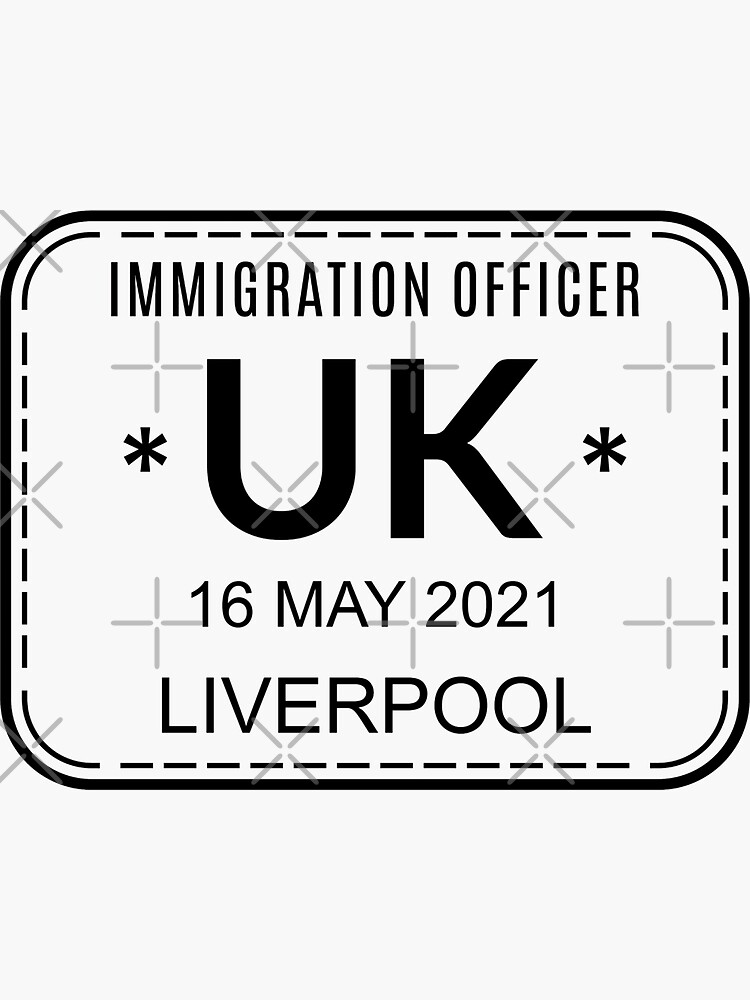This digital monochrome image features a square-like shape with rounded corners, bordered by a thin black line, and an interior perforated black border. The background is gray-white with subtle grey X's and plus signs, which may serve as watermarks. Dominantly displayed at the top in large, all-capital black letters are the words "IMMIGRATION OFFICER." Centrally located between two asterisks is "UK," followed by the date "16 MAY 2021" and the location "LIVERPOOL" inscribed near the bottom. The overall design seems to mimic a formal badge or sign.